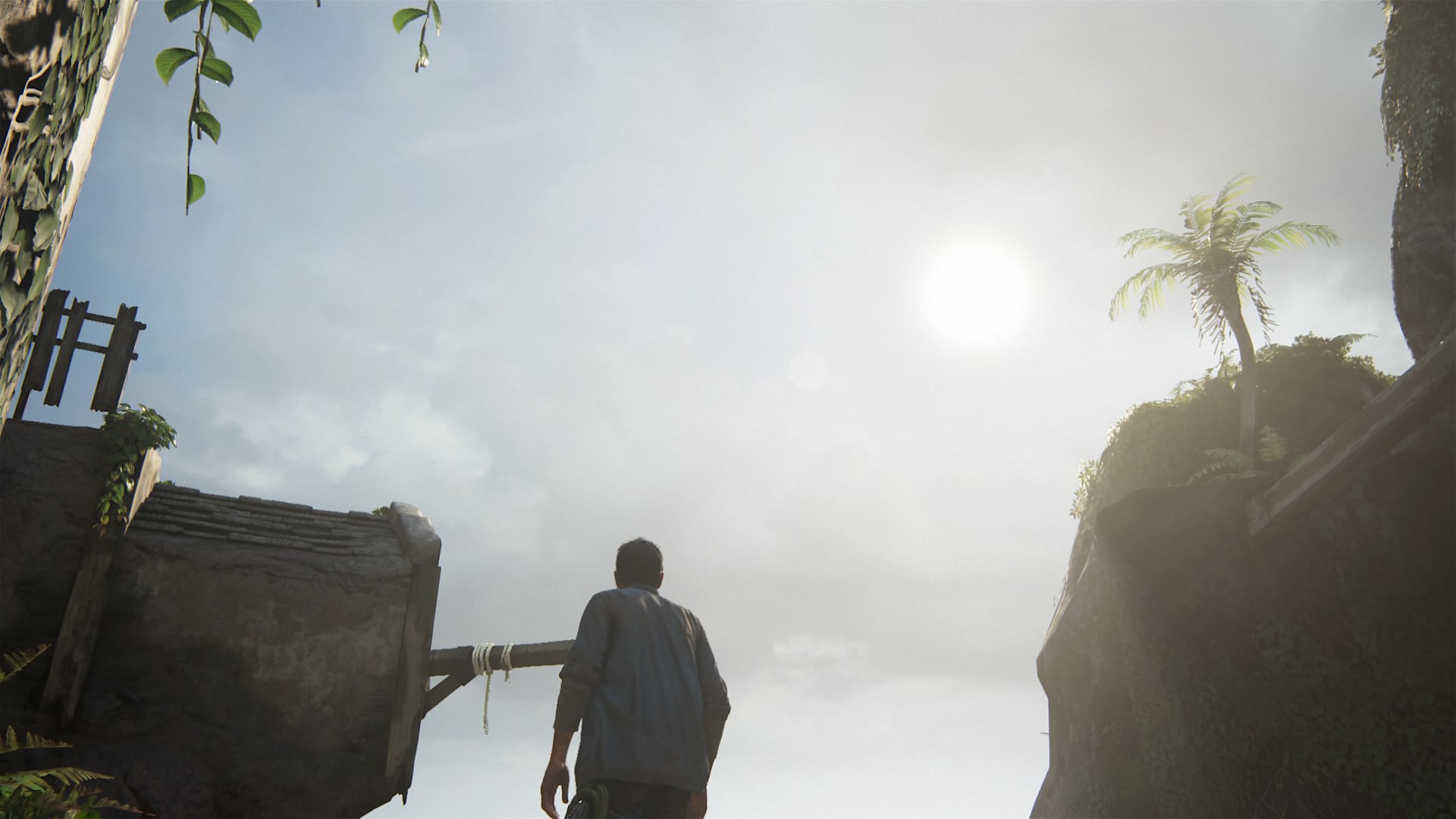In this detailed in-game screenshot, a male character stands centrally, gazing upwards into the partly cloudy, gray sky with the bright sun positioned on the top right. He has short, dark hair and is dressed in a light blue jacket and jeans, with a rope cord slung over his left side. To his left, there is a dilapidated building featuring broken stairs and a banister, with vines and vegetation creeping up its structure. Farther left, a fence, partially broken, is evident amid the overgrowth. On the right side, a small plateau rises, adorned with lush bushes and a prominent palm tree, placing the scene within a tropical setting. Additionally, branches hang down from the left side, enhancing the image's sense of depth and outdoor environment. This scene bears similarities to the visual style and thematic elements of the Uncharted video game series.